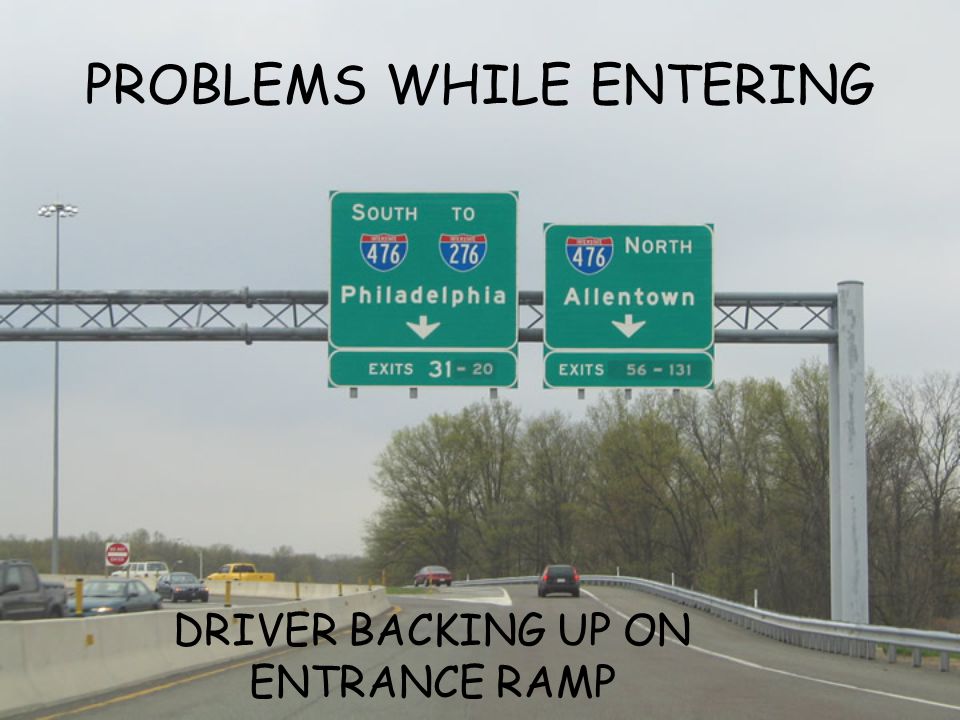This detailed image captures a bustling freeway featuring an overpass with multiple vehicles navigating through. Centrally, a prominent set of highway signs is suspended from a high pillar by a horizontal bar. The leftmost green sign directs southbound traffic with two highway shields for Interstates 476 and 276, indicating a route towards Philadelphia. Beneath these shields, white text specifies the exit numbers 31 through 20. The right sign displays a blue and red shield marked Interstate 476, guiding northbound travelers towards Allentown, with exit numbers 56 through 131. The scene also features superimposed black text: "Problems while entering" at the top, and "Driver backing up on entrance ramp" at the bottom, capturing a problematic moment on the freeway.